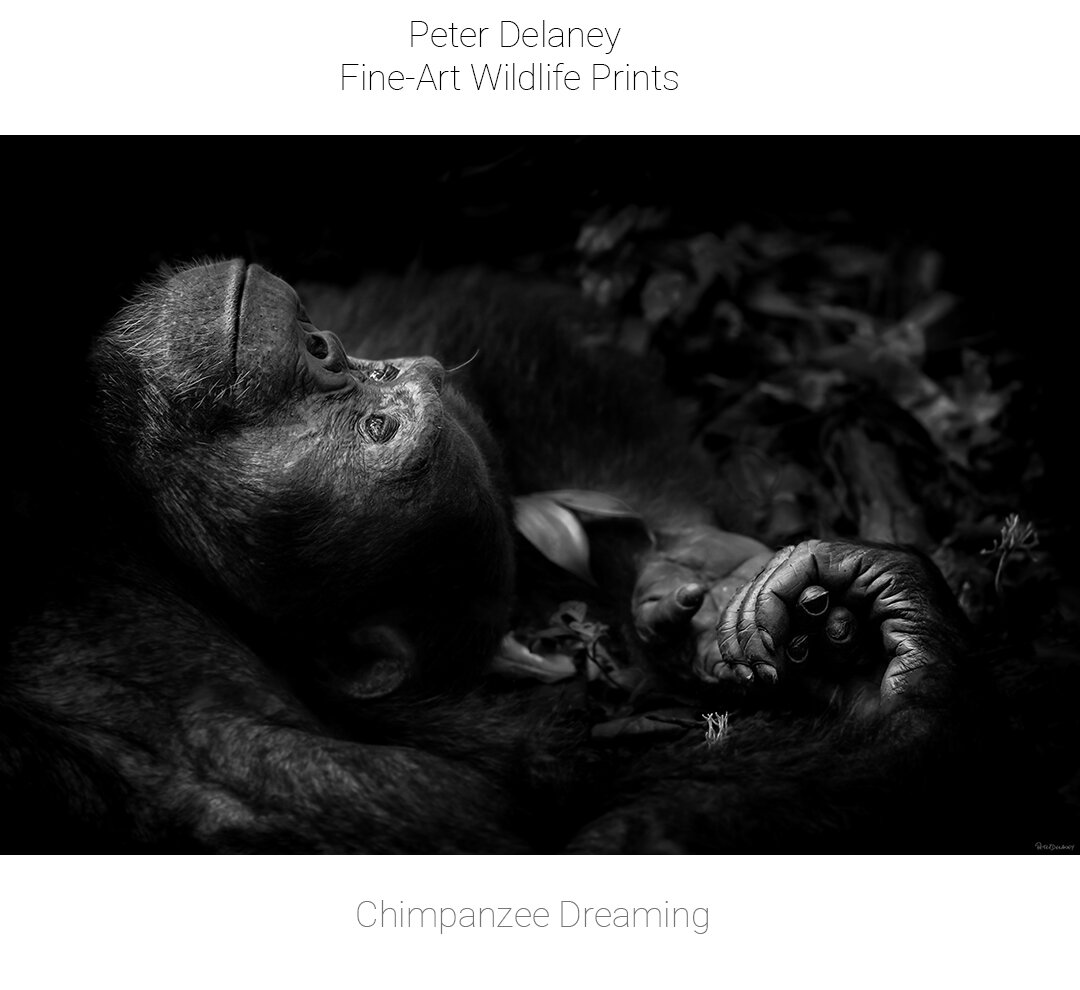This highly detailed black-and-white photograph, titled "Chimpanzee Dreaming" by Peter Delaney, captures a young chimpanzee lying on its back with its head facing upward, gazing into the distance. Illuminated by a soft light that highlights the front of its face, the chimpanzee's eyes are open, conveying a serene and contemplative expression. Its hands are positioned above its head, fingers interlocked in a clasp, which suggests an intimate connection. On the right side of the image, additional chimpanzee hands, possibly belonging to another chimp off-camera, are seen holding the visible chimp's hand. The dark background contrasts strikingly with the well-lit subject, lending a dramatic and intimate feel to the photograph, as though the viewer is laying right beside the chimp, sharing in its quiet moment.